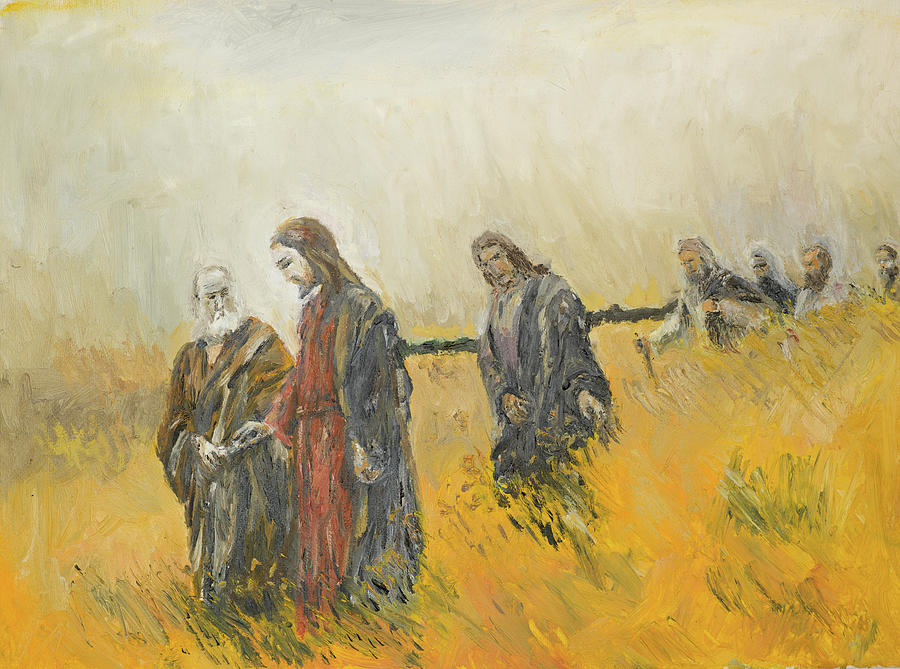The painting likely depicts a biblical scene and seems to be rendered in oil with somewhat thick brush strokes. At the forefront, there is a figure strongly resembling Jesus, dressed in a red robe with a black cloak that has tan accents. He has a beard and dark hair and appears to be looking down. Standing next to him is an older man with a white beard and hair, wearing a grayish and yellowish cloak over a tunic. This older man is looking at Jesus. Behind them, several other figures are dressed in ancient Israelite attire, including tunics and cloaks, and they appear to be walking in a line. Some of the figures trailing behind have white and gray beards and are wearing white and gray garments, adding to the sense of antiquity. There is also mention of a chain, ribbon, or cloth material linking these people together, although the exact nature of this is ambiguous. The group is moving through a field of tall, yellowish grass, possibly wheat or barley. The background features a fence or some line cutting across the landscape, and the sky transitions from grayish to white, creating a somber, almost ethereal atmosphere. Overall, the painting evokes a sense of religious significance, possibly related to Jesus Christ and biblical times.